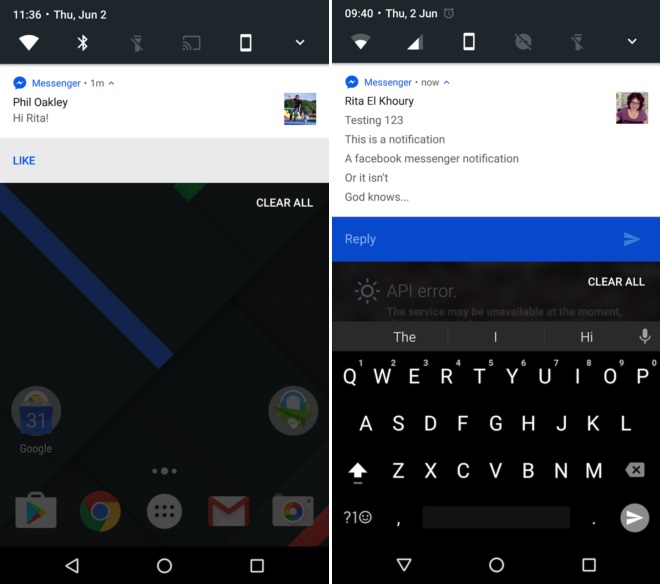The smartphone screen displays a detailed and active interface. On the top left, the time is shown as 11:36, accompanied by standard icons such as the Wi-Fi symbol, along with Bluetooth and flashlight icons that are not activated. A drop-down notification section is visible, dominated by a blue bubble with a lightning bolt icon indicating a "Messenger" notification received one minute ago.

The messenger conversation shows Phil Oakley saying "Hi" to Rita. Underneath the message, an image is present beside a gray bar with options to "Like" or "Clear All." Below this, there is information about focusing on a background that appears mostly black, with a notable blue rectangle stripe and an ellipsis (dot, dot, dot) symbol at the bottom.

In the app dock, a Google applications folder is visible, indicated by a blue rectangle labeled "Google," along with another circle likely signifying another app folder. The bottom left side of the screen displays icons for the Play Store, Google Chrome, an apps menu, Gmail, and the camera.

On the right side, a clock shows the time as 9:40 on a later date, Thursday, June 2nd. The Wi-Fi signal appears diminished, just two bars lit up. There's a Facebook message notification from Rita L. Corey, reading "Testing 1, 2, 3." Additionally, a blue rectangle hints at a service alert stating, "API or SON, the service may be unavailable at the moment." In this view, the keyboard is also shown at the bottom of the screen.